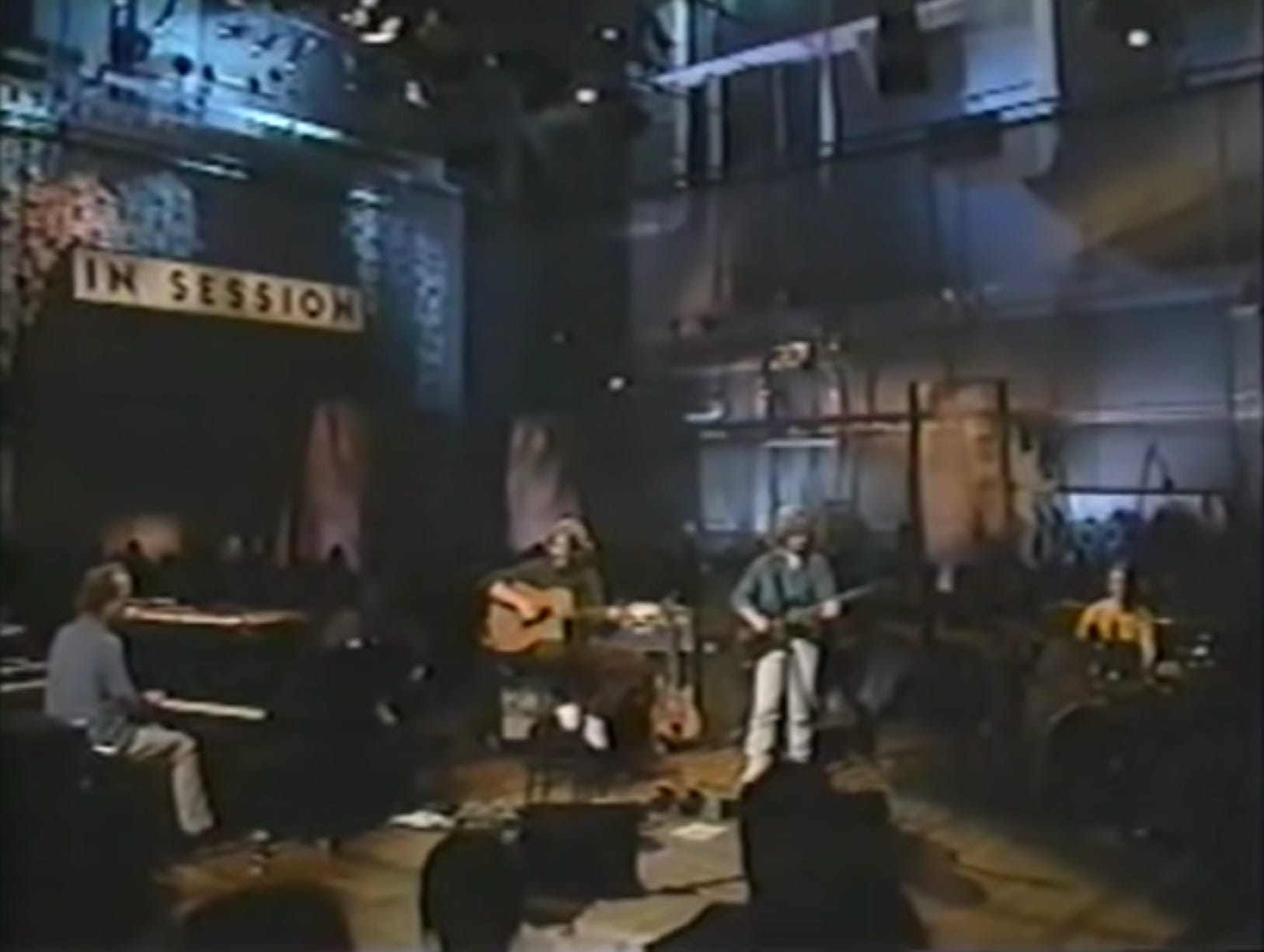In a large, dimly lit warehouse-like interior space, a band is engaged in an intimate practice session, as indicated by a prominent "In Session" sign on the wall to the left of the stage. The band consists of four members: a pianist on the far left, followed by two guitarists—one of whom is also singing into a microphone—and a drummer positioned on the far right. Amplifiers are scattered around the stage, and a mix of lighting and sound equipment dangles from the tall ceiling, illuminating the scene despite the overall darkness. The background features large metal piping and various items, adding to the industrial ambiance. The image is blurry and low-grain, making the distinct characteristics of the band members indiscernible. In the foreground, silhouettes of heads suggest a small audience observing the session. The predominant colors captured are black, gray, brown, and blue, evoking a nostalgic feel that hints at a possible 80s or retro era.